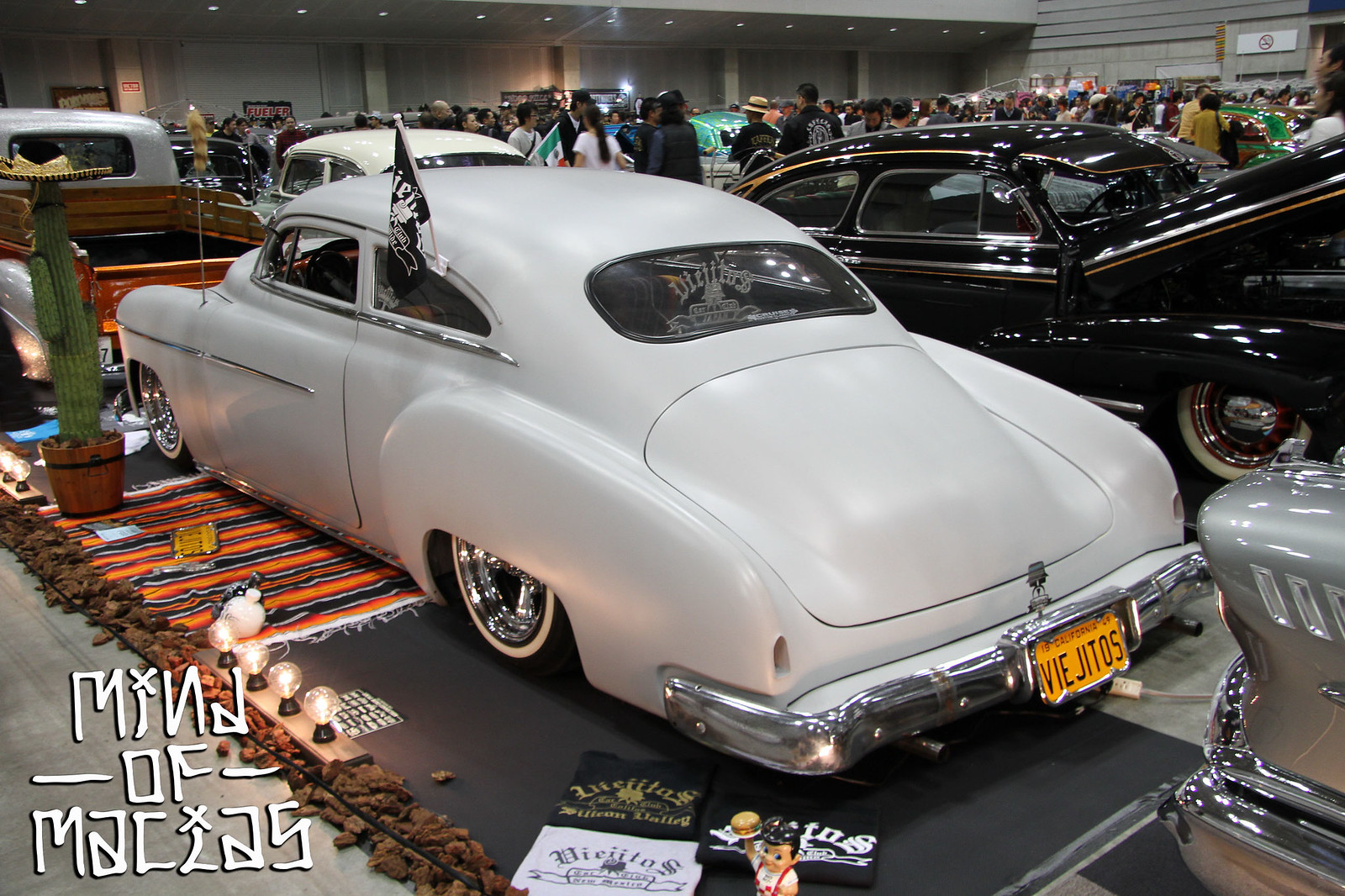This rectangular photograph captures the vibrant atmosphere of a car show, showcasing a collection of vintage vehicles in an open space. Dominating the foreground is an impeccably maintained, pearl white, 1950s-style lowrider with a sleek, curved design and shiny white wall tires. A black and white flag protrudes from the back window of this two-door vehicle, complementing its classic aesthetic. Surrounding the car is a colorful display, including an orange, black, and white Mexican-style rug, a potted cactus adorned with a sombrero, and ornamental lava rocks lining the area.

To the right of the white lowrider stands a gleaming black vehicle with intricate golden lines and an open hood, adding to the exhibition's allure. Partially visible in front of the white car is the rear end of an antique pickup truck, featuring an orange-gold and white color scheme and a vintage wooden bed. The space beyond these cars is bustling with people who meander around, admiring the various automobiles.

In the background, a blend of concrete structures and rows of vintage cars — mainly from the 1950s lowrider genre — can be seen. Scattered among the display are magazines and possibly t-shirts. The bottom left corner of the photo features white handwritten text that reads "MIND MACIAS," with the letters "I" and "A" printed backward, adding a quirky element to the scene.